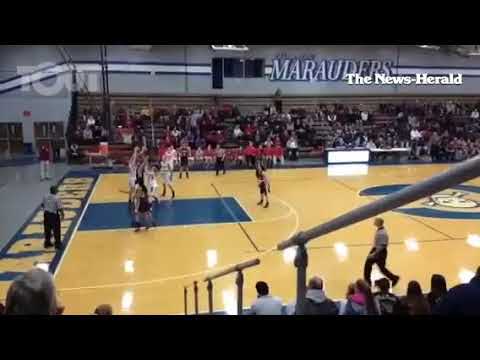The image captures a lively basketball game, likely in a high school or college gymnasium. Taken from the middle or upper section of the stands, the viewer looks across the court from a vantage point on the long side of the court, closer to the left end. The court displays classic wooden tones, with the field goal area and center logo highlighted in blue. Prominent on the opposite side is a wall adorned with thick white and thinner blue stripes, displaying the name "Marauders" in bold white letters with a blue outline, aligned at what appears to be the half-court mark. Overlaying this background is the watermark or header text reading "The News-Herald."

The scene shows two referees, one positioned past the rim on the far left, and another moving in from half-court. Below the latter, a bench crowded with people, possibly team substitutes in red uniforms, is visible. In the stands behind them, rows of spectators are watching the game intently. At the moment of the shot, most players are positioned below the rim, with one player appearing to take a free throw, hinting at a potential foul situation. The picture captures the dynamic atmosphere of the game, with layers of onlookers and athletic action.